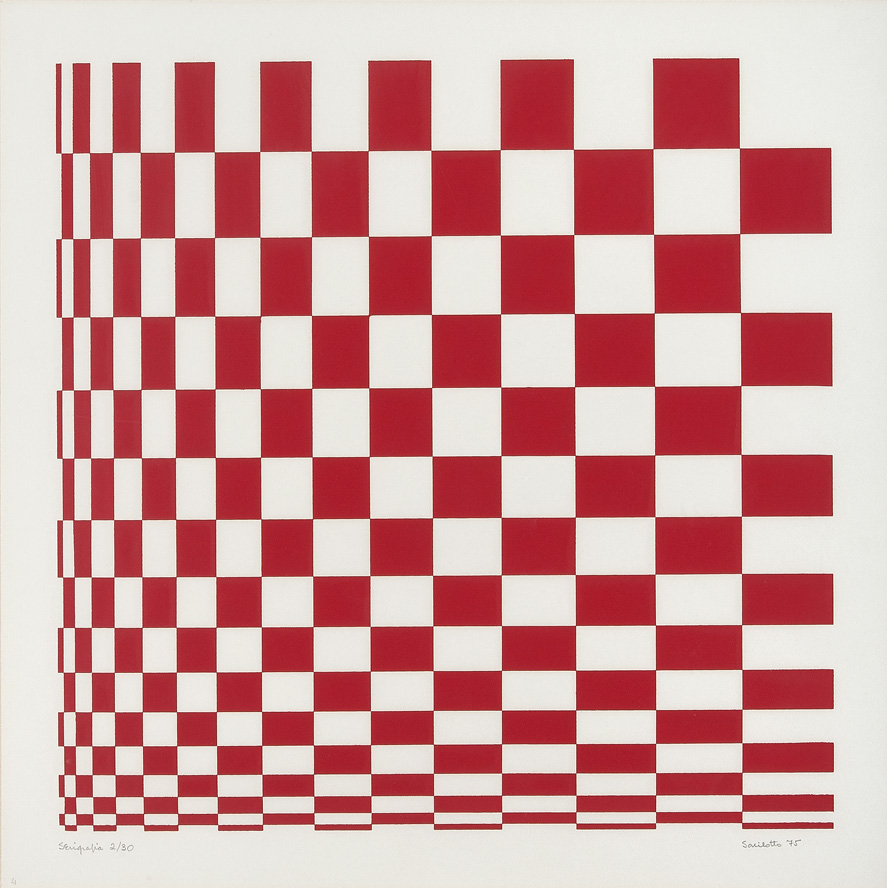This image is a detailed, abstract art piece resembling a red and white checkerboard set against a white background. The upper right section of the image features standard, alternating red and white squares. As you move towards the bottom left corner, the squares progressively shrink and morph into increasingly thin rectangles, creating a striking optical illusion of curvature. The bottom left corner culminates in minuscule squares that give the impression of a distorted and compressed pattern, enhancing the sense of depth and complexity. Notably, there are signatures marked "220" on the bottom left and "95" on the bottom right, adding an element of intrigue to the piece. The meticulous arrangement and gradual transition of shapes evoke a mesmerizing, almost Escher-like visual experience.